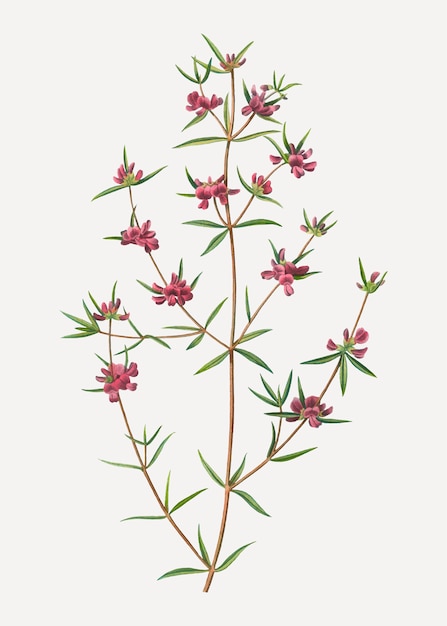The image showcases a delicate painting of a plant with thin, brown stems and sparse clusters of small flowers and leaves on a plain white background. The central vertical stem extends upward, with several smaller branches protruding from both sides at various points. These branches curve gently upwards, leading to clusters of small, vibrant red flowers and long, slender green leaves. The flowers, found mainly at the ends of the branches, vary in their stages of bloom—ranging from tiny buds to fully opened petals—yet all remain modest in size. The overall composition highlights the plant's fragility and elegance against the starkness of the white paper.